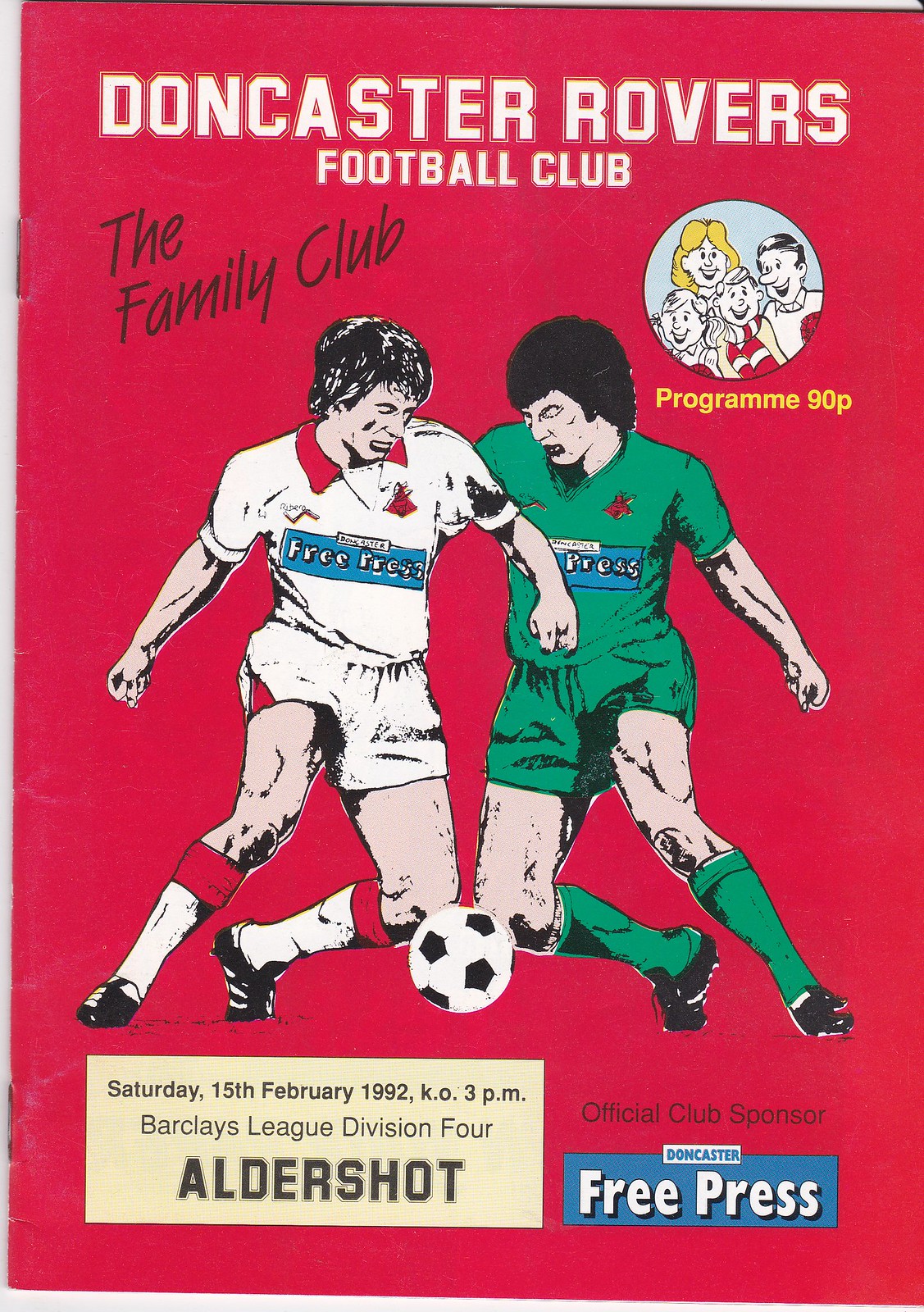The cover of the program for Doncaster Rovers Football Club prominently features the title "Doncaster Rovers Football Club" in white font at the top, with "The Family Club" in black print slightly to the left below it. The main image showcases two players from opposing teams vying for a black and white soccer ball. The player on the left is dressed in a white jersey, white shorts, and red and white socks, while the opposing player on the right is outfitted in a green jersey, green shorts, and green socks. Both players are wearing black cleats.

Below this image, text details the match date as "Saturday, 15th February 1992" with a kickoff time of "3 p.m." for a Barclays League Division 4 game against Aldershot. The information is in white font positioned in the lower left. To the right, it states "Official Club Sponsor" and "Doncaster Free Press" against a blue background. In the upper right corner, a circular emblem contains a caricature of a smiling family - a man, a woman, and two children. The program is priced at 90 pence, indicated within or near this circle.